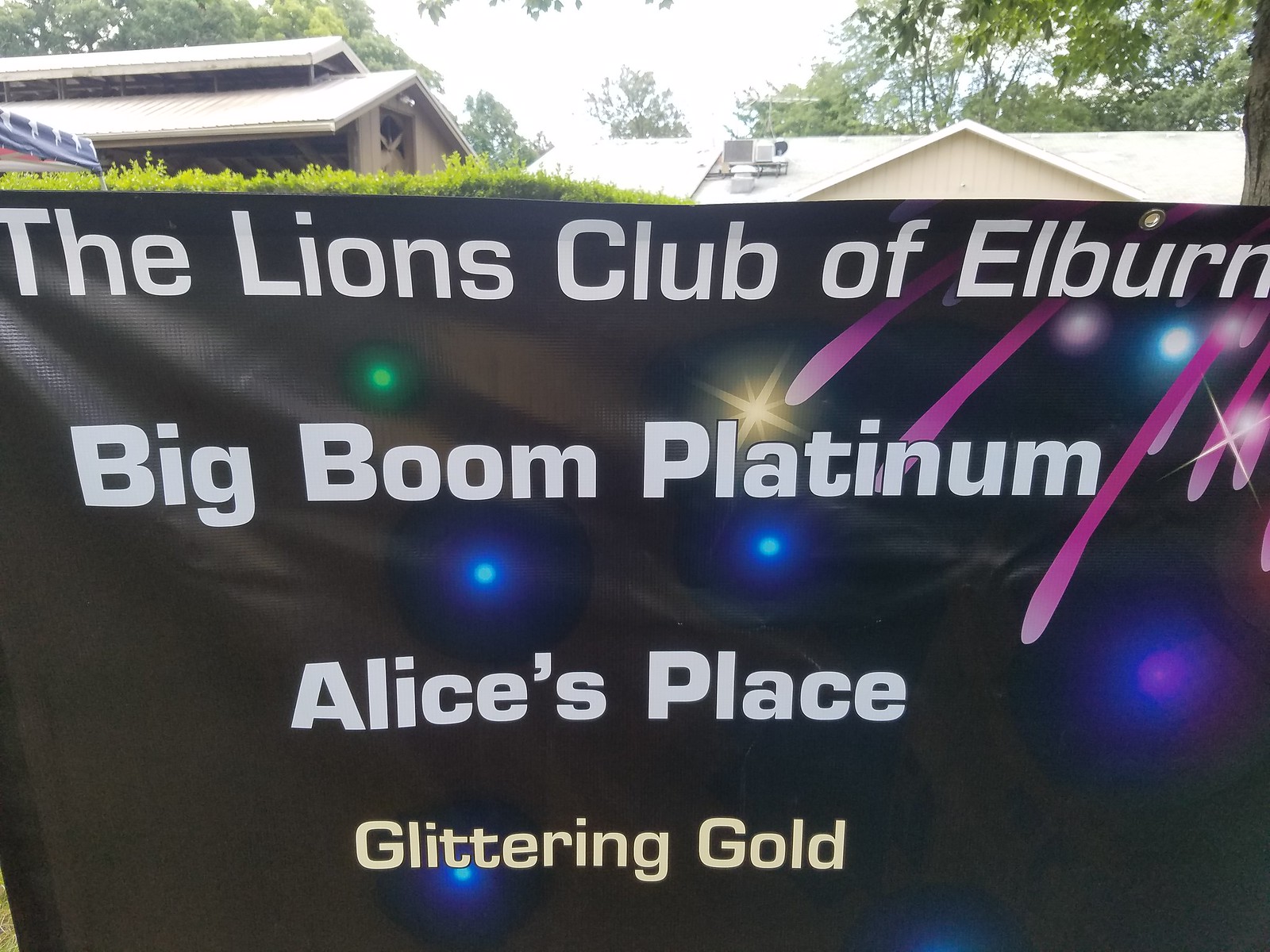This photograph captures a detailed view of a black banner, seemingly hanging from a window, with a backdrop of a suburban area. The banner prominently displays white text, starting with "The Lions Club of Elburn" at the top, followed by "Big Boom Platinum" in larger letters in the center, "Alice's Place" beneath it, and "Glittering Gold" at the bottom in a gold-colored font. The banner features a variety of lights and designs: blue circular lights in the center and lower left, a solo green light towards the top left, and streaks of purple descending from the upper right corner towards the center. There are also pink falling star-like designs. In the background, the bright daylight casts a white hue on the sky, revealing the roofs of houses and other buildings with triangular shapes. These structures are surrounded by lush green trees, all set against a clear, light blue sky. This scene likely suggests a promotional sign for an event hosted by the Lions Club of Elburn.